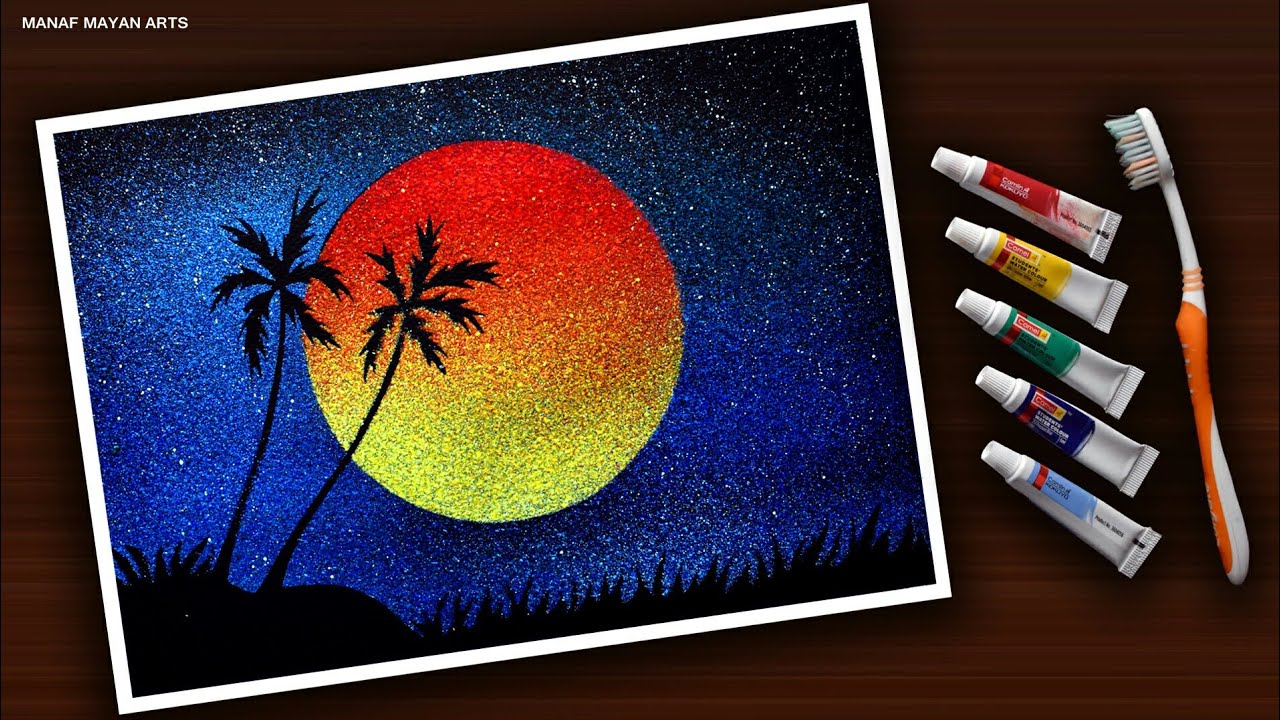The image features a detailed artwork prominently displayed on the left side, with a striking dark brown, wooden-textured background. The artwork itself is encased in a white-bordered rectangular frame, creating a postcard-like appearance. At the top left corner, the words "MANAF MAYAN ARTS" are inscribed. The centerpiece of the artwork is a circular object with a vertical gradient transitioning from red at the top to yellow at the bottom, evoking the image of a sun or moon. Surrounding this circle is a dark blue sky, adorned with white dots resembling stars. Silhouettes of palm trees are seen against this celestial backdrop, with one tree’s silhouette partially crossing the glowing circle. Below, there is a black landscape with the silhouettes of grass. 

To the right of this picturesque artwork, five paint tubes are arranged in a vertical line. From top to bottom, the tubes display locations of vibrant colors: red, yellow, green, dark blue, and light blue, although each tube is primarily white with a splash of its respective color. Each tube has illegible writing on it. Further right of the paint tubes lies an orange and white-handled toothbrush. The entire composition gives a sense of a creative workspace, juxtaposing artistic tools against a sophisticated wooden background.